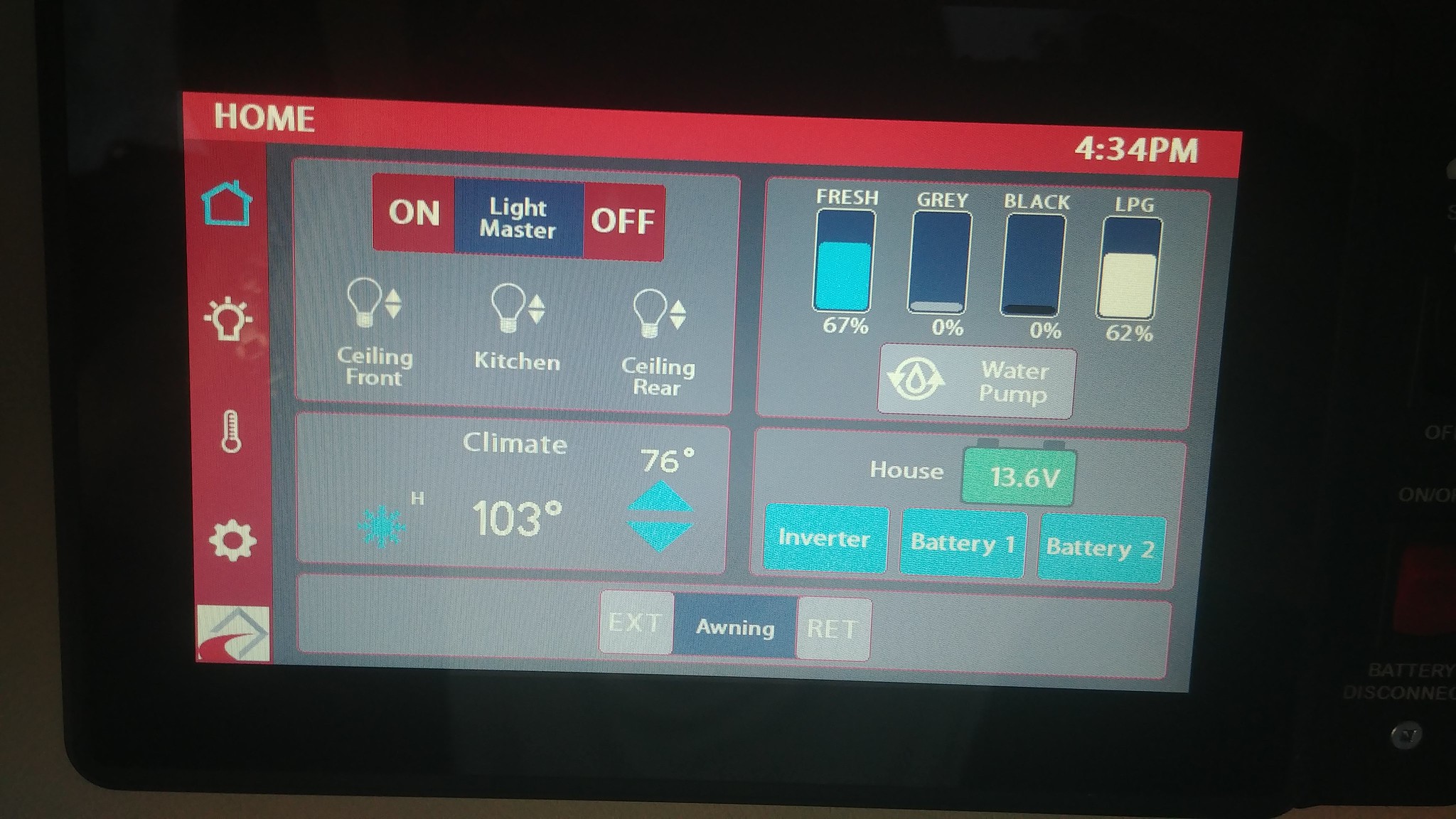The image features a user interface with a complex and detailed control panel, primarily designed in a color scheme that includes black, brown, red, blue, gray, and white elements. On the left side, the background transitions from black to brown, creating a gradient effect. This area includes a red rectangle, labeled "Home," and adjacent to it, the time "4:34 PM" in bold text. Beneath the "Home" label is another red rectangle, inside of which are icons: a blue house, a white light bulb, a white thermometer, and a white settings symbol.

Below this section, the background turns white and displays a segment of a blue square intersected by a red wave. There is also a dark blue rectangle containing a light blue rectangle, outlined thinly in red. Further down is a red square stating "ON" in white text, a blue rectangle labeled "Light Master" in white, and another red rectangle marked "OFF" in white.

The interface further details three light bulb icons accompanied by arrows pointing up and down, labeled "Ceiling Front," "Kitchen," and "Ceiling Rear" respectively. Underneath these controls lies a gray rectangle, thinly outlined in red, with the word "Climate" in white. Adjacent is a blue star symbol followed by the letter "H," and temperature readings of "103 degrees" and "76 degrees" with arrows indicating adjustment options.

To the right is another gray rectangle, also outlined in red, featuring a dark blue and light blue rectangle indicating "Fresh: 67%." Adjacent labels include "Gray: 0%" with blue and gray tones, "Black: 0%" with blue and black, and "LPG: 62%" in blue and cream hues.

A lighter rectangle, thinly outlined in red, is labeled "Water Pump" with a circular symbol featuring two arrows and a drop icon. Additional controls include another gray rectangle outlined in red marked "House." A green rectangle, outlined in blue, displays "13.6V" in white with two small blue caps. Blue rectangles labeled "Inverter," "Battery 1," and "Battery 2" are also present.

At the bottom, a gray rectangle outlined in red contains a light gray outlined square with barely visible text "EXT" against a light gray background. Lastly, a blue rectangle outlined in red is labeled "Awning," followed by another blue square outlined in red, marked "RET."